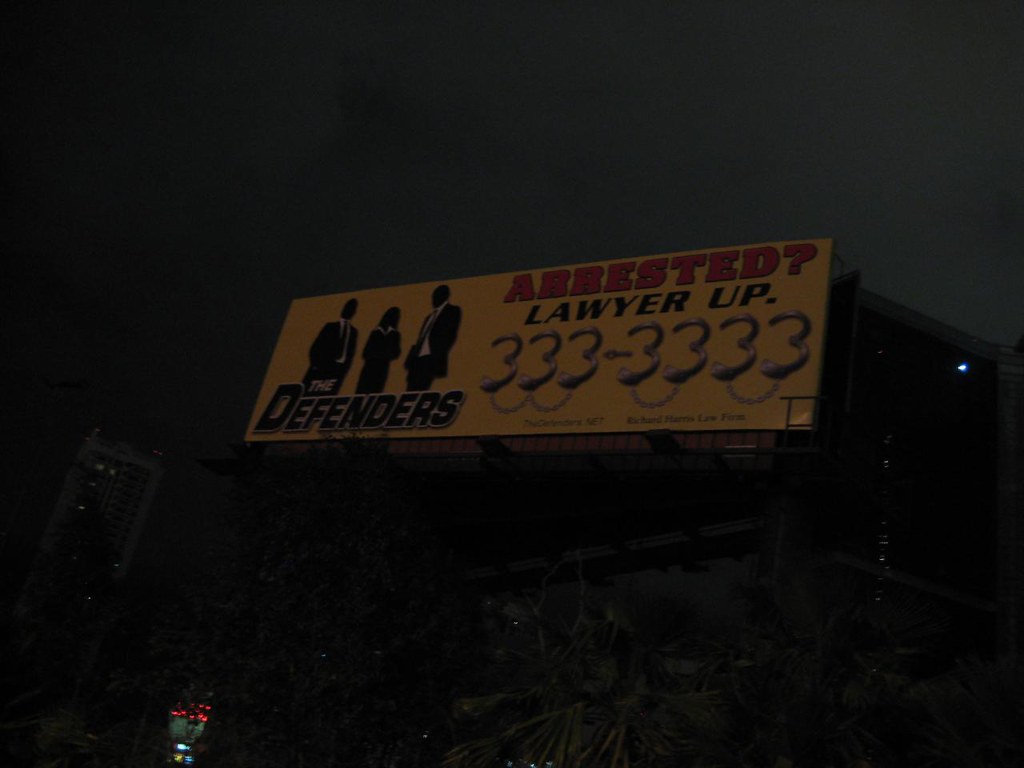The image is a dark, outdoor photograph of a rectangular billboard. The billboard has a skewed yellow background and features three silhouetted figures in formal attire; two men in suits flank a central figure appearing to be a woman in a dress, all with blacked-out faces. The word "Defenders" is written below the figures in bold, shadowed black letters with a white border. At the top right of the billboard, "ARRESTED?" is prominently displayed in big, bold red capital letters with a subtle black border. Directly beneath, "LAWYER UP" is italicized and bold in black capital letters. The contact number "333-3333" is written in gray, with the bottom curves of the threes linked together by illustrations resembling barbed wire or handcuffs. The billboard also includes metal lines indicating its structural support, and buildings bordered in gray can be seen on either side of it.